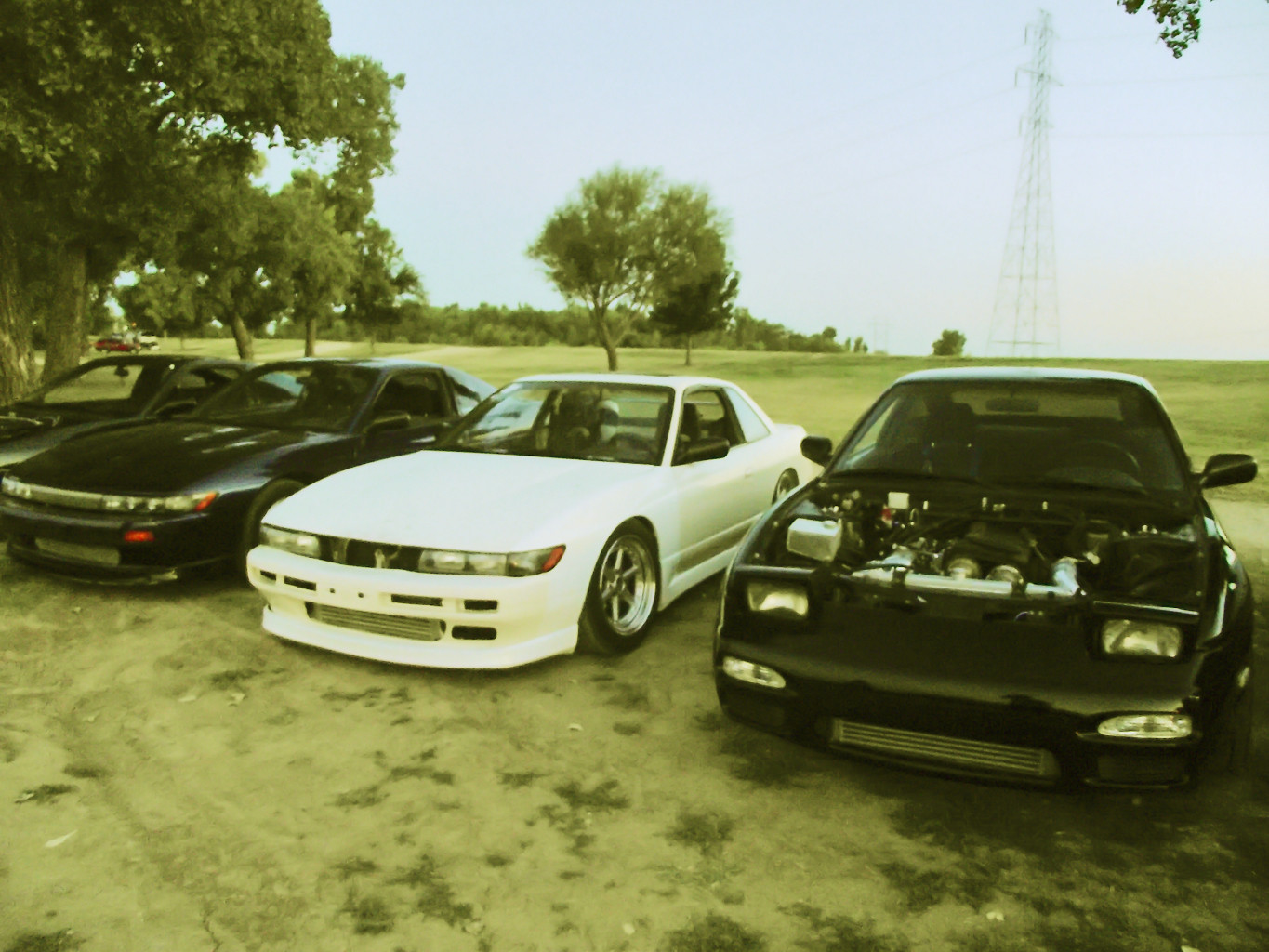This image captures a serene, overcast day in what appears to be a large, grassy field, framed by the green hues of trees and an imposing electric tower in the background. The sky is a muted gray-blue, heightening the tranquil atmosphere. Four cars are aligned horizontally across the field, drawing attention with their classic, old-school aura. The car closest to the right of the photo is a black car, notably lacking its hood, exposing its intricate internal mechanics. Moving leftward, a white, low-to-the-ground car, possibly a Nissan Silvia, stands with its windows down. Next, another black car with its windows down sits poised on the grass, followed by a partially visible black car further left, partially obscured by the edge of the photo. In the distant background, a red car can be seen parked, adding a splash of color to the predominantly green and gray scene. This well-crafted composition blends the nostalgic charm of vintage cars with the calm of the natural setting.